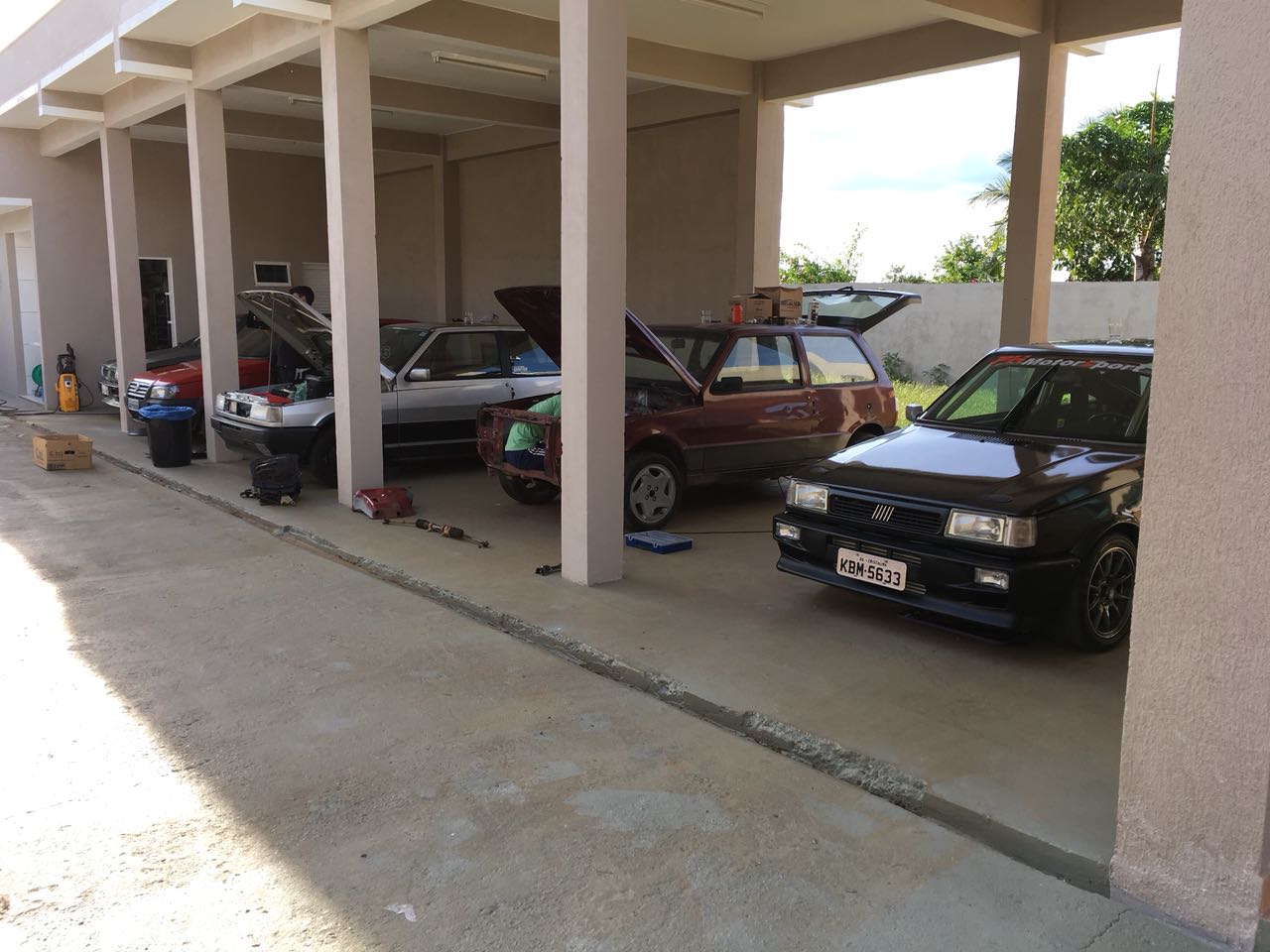This digital photo showcases a home carport, likely situated in a warm, tropical environment, possibly Florida. A washed-out white sky serves as the backdrop, accompanied by a cinder block wall with a strip of grass and several trees, including palm fronds, hinting at the subtropical climate. The focal point is a white-roofed carport with beige pillars, open at the front and back, housing four older model vehicles parked on a grey concrete floor. 

Two of the cars, a silver one and a red one bearing the license plate "KBM 5633," have their hoods raised, indicating ongoing repair work. The red car also has its trunk open. One of the cars, a burgundy or orange-red hue, has a person wearing blue shorts and a green or yellow shirt sitting inside, suggesting it lacks an engine. Another car, a black one, appears parked with tools and boxes scattered around. Various miscellaneous tools and cardboard boxes are seen around the workspace, adding to the atmosphere of a makeshift repair garage.